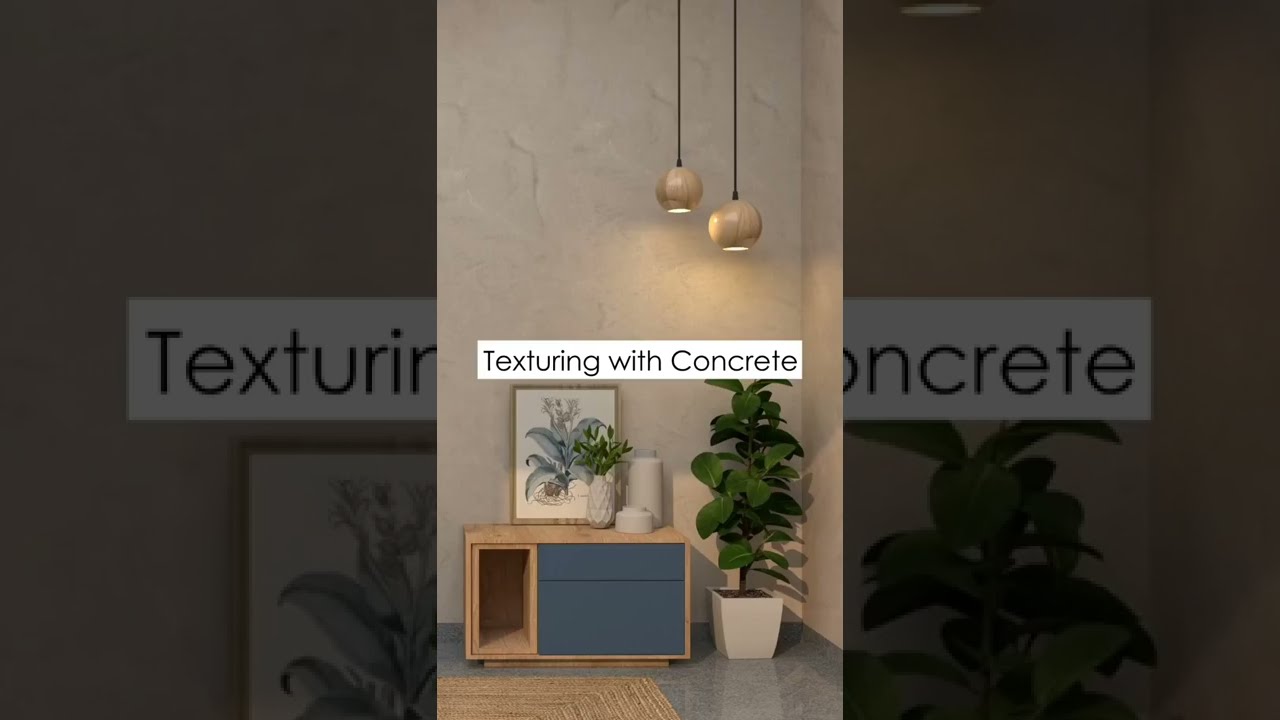The image features a sophisticated, minimalist room with a light gray textured wall and polished grayish flooring. Dominating the scene is a small wooden table with blue drawers, one of which is slightly open. This table is positioned on what appears to be a corner of a fancy, dried grass rug. On top of the table, there is a white vase containing green flowers, flanked by two additional white decorative objects, and a propped-up artistic picture of a flower.

To the right of the table stands a tall potted house plant with lush green leaves in a white planter. Hanging above the scene, there are two modern, sphere-shaped tan overhead lamps made of wood. The photograph is overlaid with a banner that reads "texturing with concrete" in black font on a white rectangular background. The central image is set against a darkened, larger duplicate of itself, providing a layered visual effect.